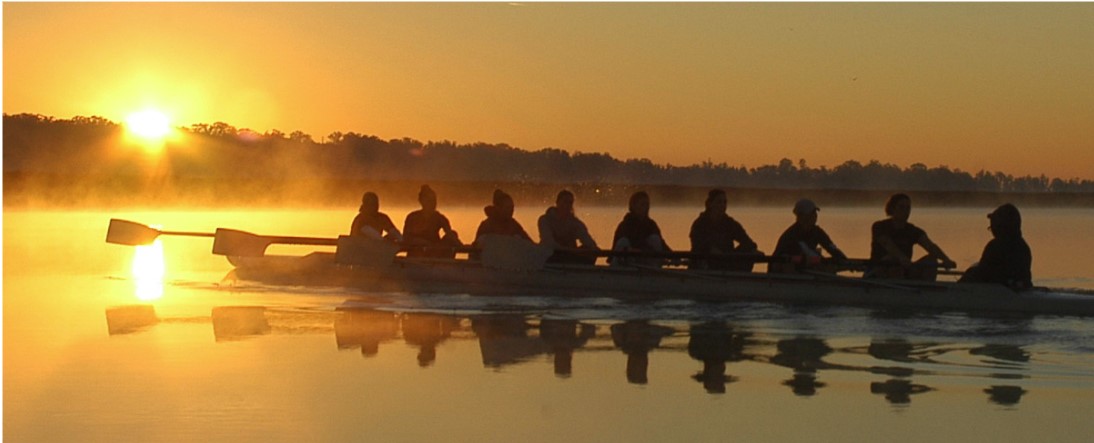This photograph captures a rowing team gliding across a serene lake at dawn. The team is composed of eight rowers, each equipped with an oar, and a coxswain at the front of the boat, who faces the rowers to guide and oversee their practice. The rowers, mostly clad in hoodies, appear as shadowy silhouettes due to the bright, rising sun behind them. The sun, a dazzling white-yellow orb, illuminates the sky in gradients of gray, orange, yellow, and deep brown, creating a striking backdrop. The calm water perfectly reflects the boat and its occupants. In the background, the shoreline features low hills adorned with trees that stretch across the horizon, adding to the tranquil and picturesque scene. The absence of uniforms suggests this is a practice session, highlighted by the stillness of dawn and the natural beauty surrounding the team.